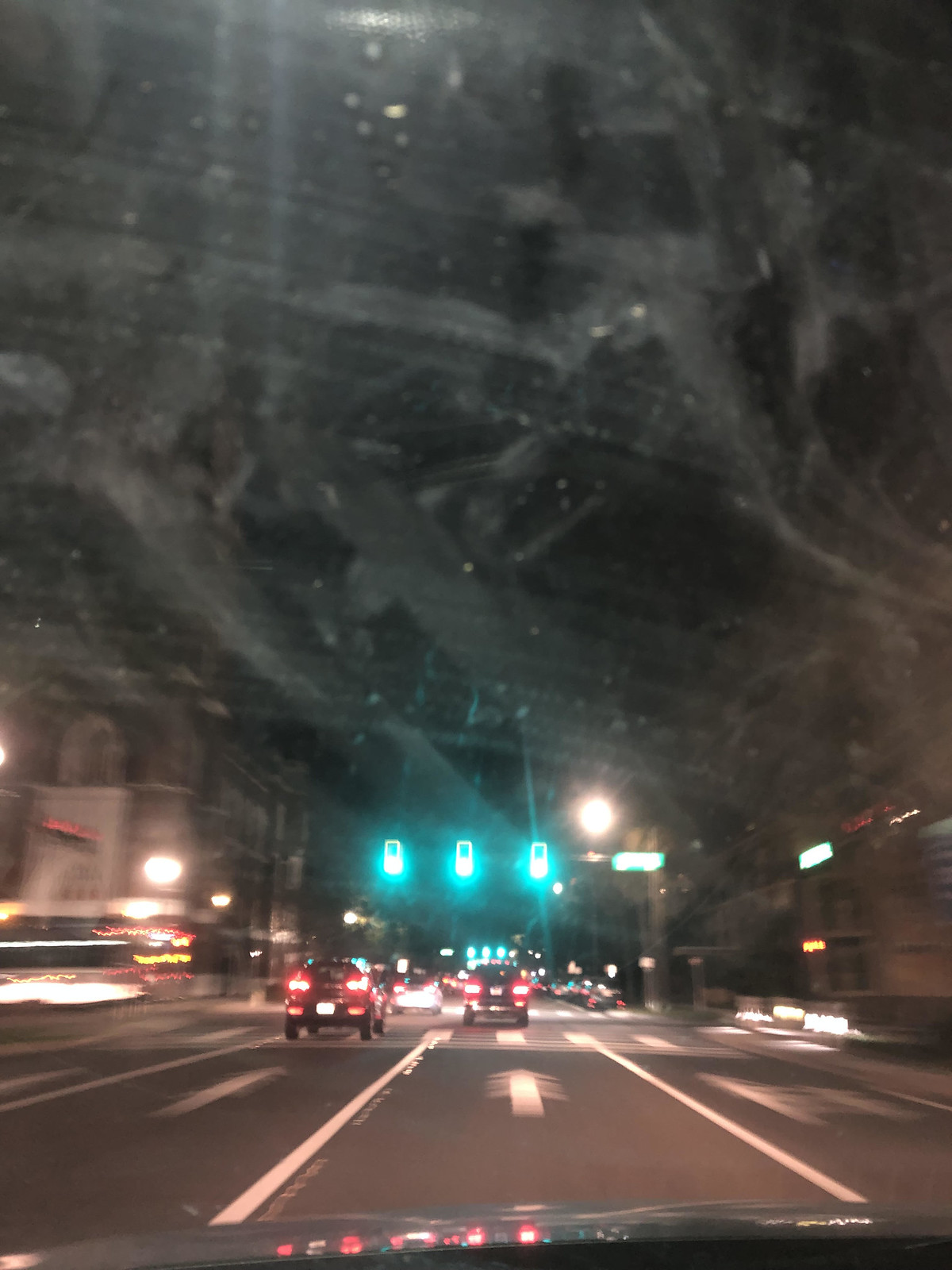This nighttime photograph, taken from inside a moving car in the middle lane, captures a city street through a dirty and streaked windshield. The image prominently features the car's gray hood in the foreground and displays significant motion blur, suggesting the vehicle is in motion. The road, which consists of at least three or four lanes running in the same direction, is marked with white lines and arrows. Ahead, the blurry outlines of other cars can be seen with their brake lights glowing red. Green traffic lights are both directly above and further down the road, indicating the car is approaching an intersection, possibly with a three-way stop, just under an overpass or bridge. To the left, a brick building with white doors and trim is barely visible, while on both sides of the scene, various red, green, and yellow lights add to the urban ambiance, hinting at the presence of shops or small businesses. Overall, the photograph gives a somewhat chaotic and congested impression of a city street at night.